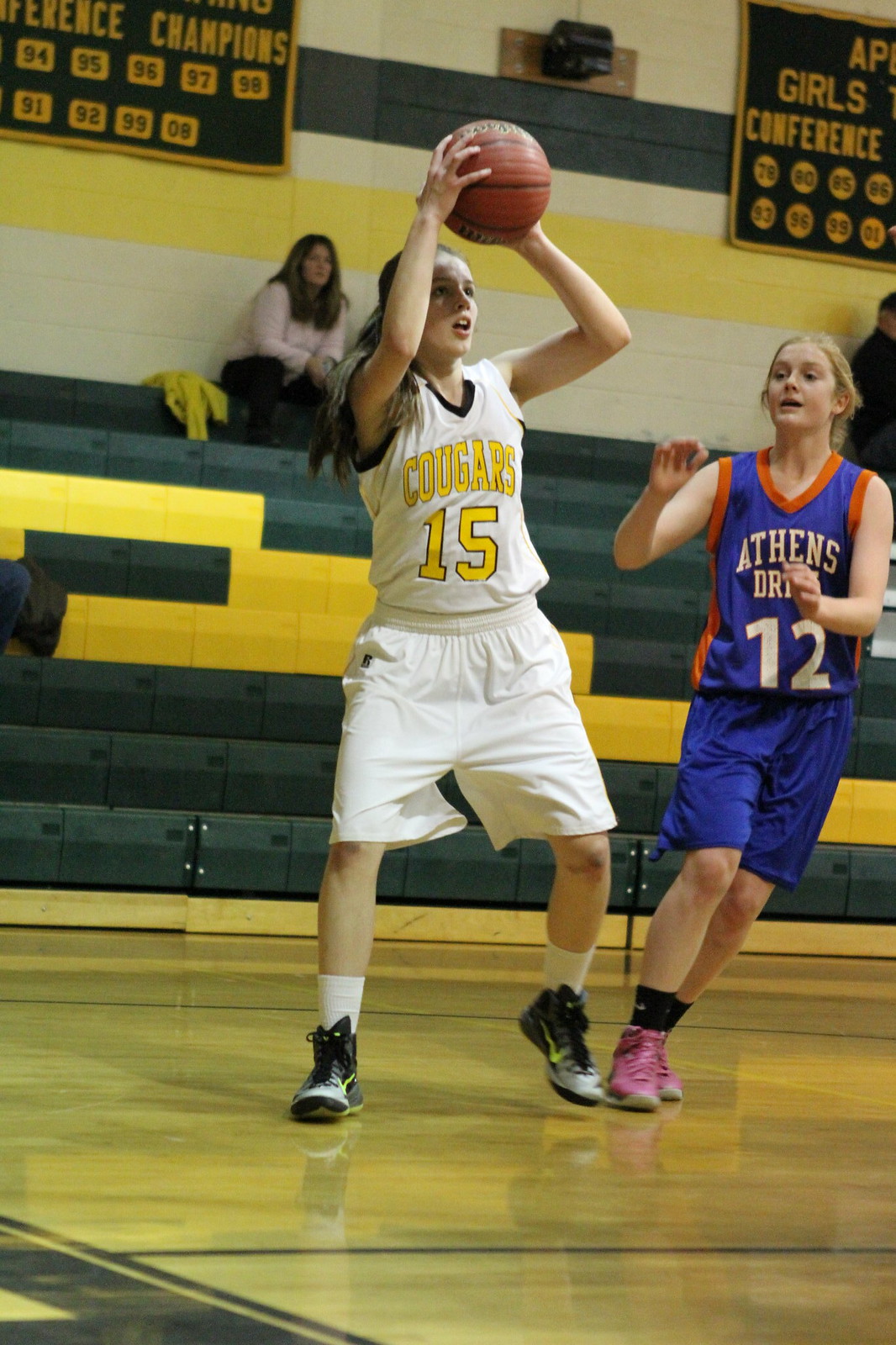The photograph captures an intense moment of a basketball game between two girls from opposing teams set against the backdrop of a gymnasium. The girl on the right, dressed in a white jersey emblazoned with "Cougars" and the number 15 in yellow, has her long brunette hair pulled back and appears to be aiming a shot with the basketball held above her head. She is outfitted in matching white shorts, white socks, and black Nike shoes. Directly next to her, attempting to block the shot, is a blonde girl in a bright blue jersey with orange trim that reads "Athens" and the number 12. She complements her uniform with blue shorts, black socks, and pink shoes. The basketball court gleams with its polished wood plank flooring, marked by black lines. In the background, the bleachers feature a distinctive green and yellow zigzag pattern and host a few spectators. The walls are painted in a combination of white, yellow, dark green, and cream, adorned with partially visible dark green and gold banners. The image is a vibrant depiction of youthful athleticism and competitive spirit in a minimally crowded gym.